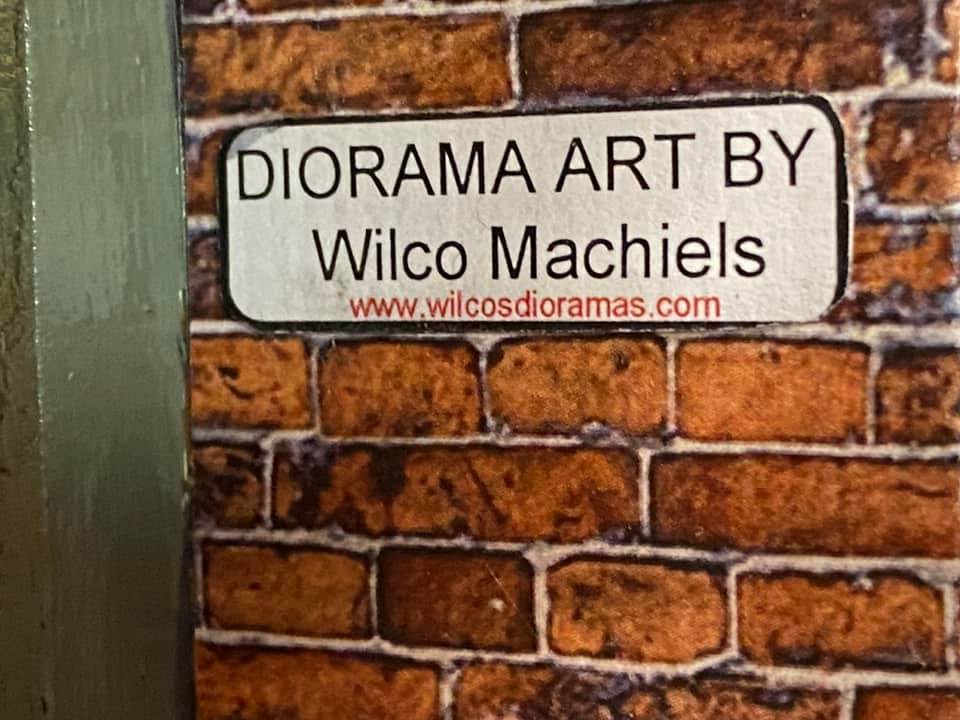The image appears to be a digital rendering rather than a photograph, depicting a brown brick wall with visible white grouting. On the left side of the image, there's a vertical piece of wood painted dark green. Near the center of the wall, towards the upper part of the image, a white rectangular sign with rounded corners and a black border is prominently displayed. The sign reads in black capital letters "DIORAMA ART BY," followed by "Wilco Machiels" with capitalized initials. Below this text, the website "www.wilcosdioramas.com" is printed in red.